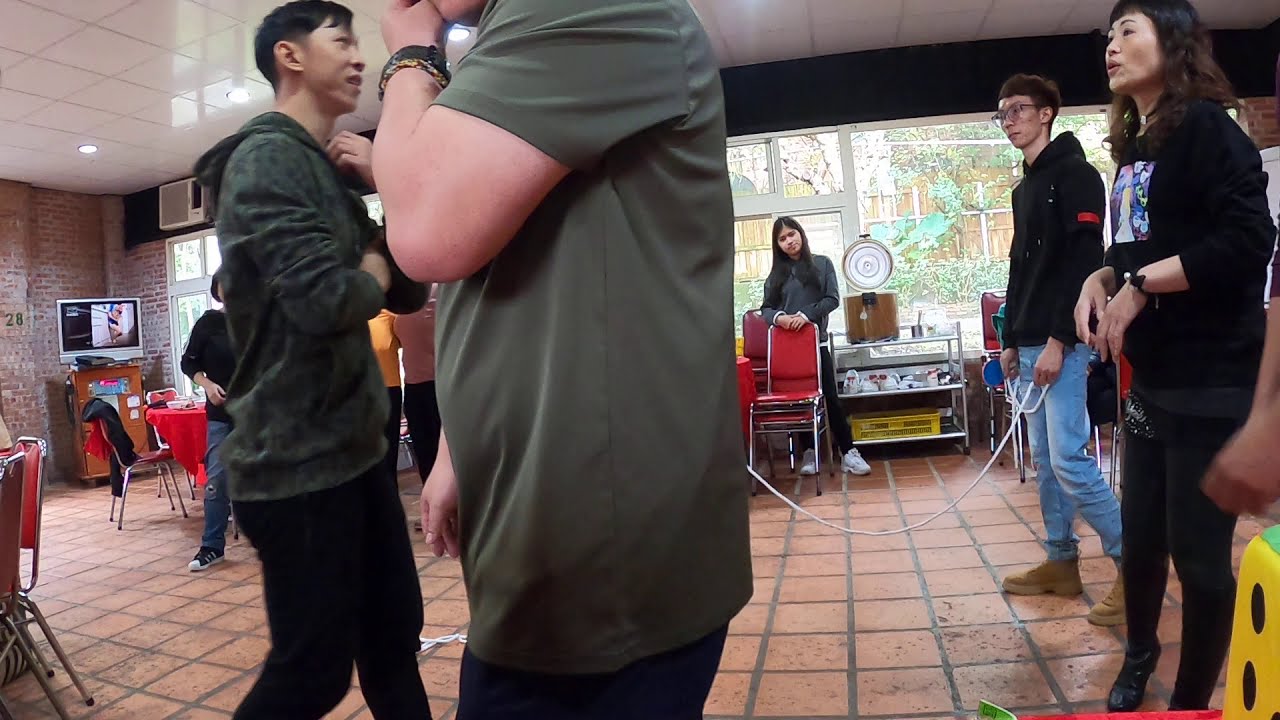This color photograph captures a bustling scene inside a restaurant with light orange terracotta tiles and gray grout. Prominently in the foreground is a man in a green shirt and black pants, facing left, his arm bent as he touches his face. To his left stands an Asian man wearing a hoodie and black pants, characterized by his short black hair just touching his forehead. On the right side, an Asian woman with shoulder-length hair dons a black sweatshirt featuring a square with a unicorn in purple, pink, and white, and black pants. Beside her, towards the back, is a man in a black hoodie, white-blue jeans, brown work boots, short brown hair, and glasses. Further in the distance, behind a red chair, a person with middle-parted hair down to her shoulders and clad in a gray long-sleeve shirt, black pants, and white shoes stands. The scene includes red chairs, and the back wall features a window with white framing, showcasing a wooden fence and green vegetation outside. The white tile ceiling reflects light, adding brightness to the space. The far left wall stands out with its exposed brick and white concrete, marked by the number 28, and a silver-framed TV rests on a wooden shelf below. This vivid setting suggests a communal space filled with diverse individuals, possibly Asian youth, engaging in various activities.